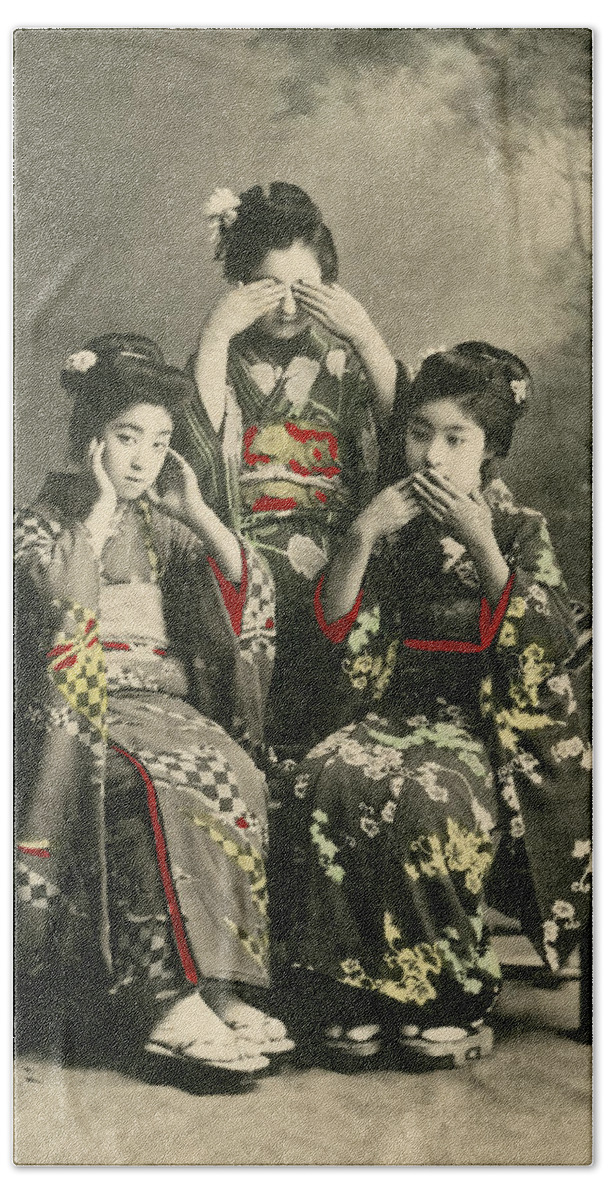This is a vintage, partially colorized photograph of three Japanese children, likely girls, dressed in traditional kimonos. The image, predominantly black and white with selective color enhancements, depicts the children arranged in a triangular formation – two seated in the foreground and one standing between them. They embody the "see no evil, hear no evil, speak no evil" concept through their hand gestures: the girl on the left covers her ears, the standing girl in the middle covers her eyes, and the girl on the right covers her mouth.

The kimonos feature three distinct patterns: checkered, floral, and large floral prints. The added color highlights elements of their attire, showcasing bright red lines on the kimonos and a red sash with floral patterns around the waist of the girl in the middle. Additionally, some flowers appear in yellow, likely part of the original design.

The background is a grayish wall with a faintly discernible tree silhouette on the right side, contributing to the image's aged, slightly yellowed appearance. The overall composition and the partially colorized elements emphasize the cultural and historical significance of the traditional Japanese garb and the timeless message of the "three wise monkeys."